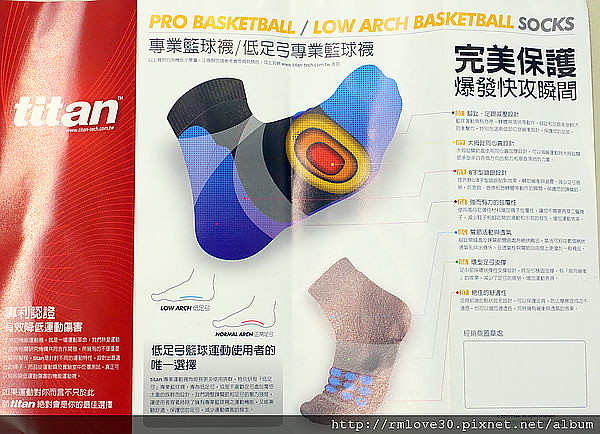The image showcases a detailed promotional advertisement for specialty basketball socks. Dominating the layout, the product packaging occupies almost the entire frame with vibrant and contrasting colors. The left vertical one-fourth of the image features a striking red column with dynamic yellowish glowing lines and the word "Titan" prominently displayed in large white letters. Beneath "Titan," there is a cluster of Chinese or Japanese text.

The top section of the image displays the phrases "Pro Basketball, Low Arch, Basketball Socks" in gold letters set against a yellowish-green background. Central to the image, a sizable blue sock is illustrated with an intricate design showing internal layers transitioning in color from yellow to red, indicating heating zones. Below, there is another image of a pinkish-gray sock adorned with blue dots around the arch area.

Further details about the product's features are listed on the right side, with lines connecting each description to specific parts of the sock. The advertisement's color palette includes hues of red, off-red, white, gray, black, blue, light blue, yellow, and tan. The composition effectively highlights the socks' innovative design and functionality aimed at basketball players.